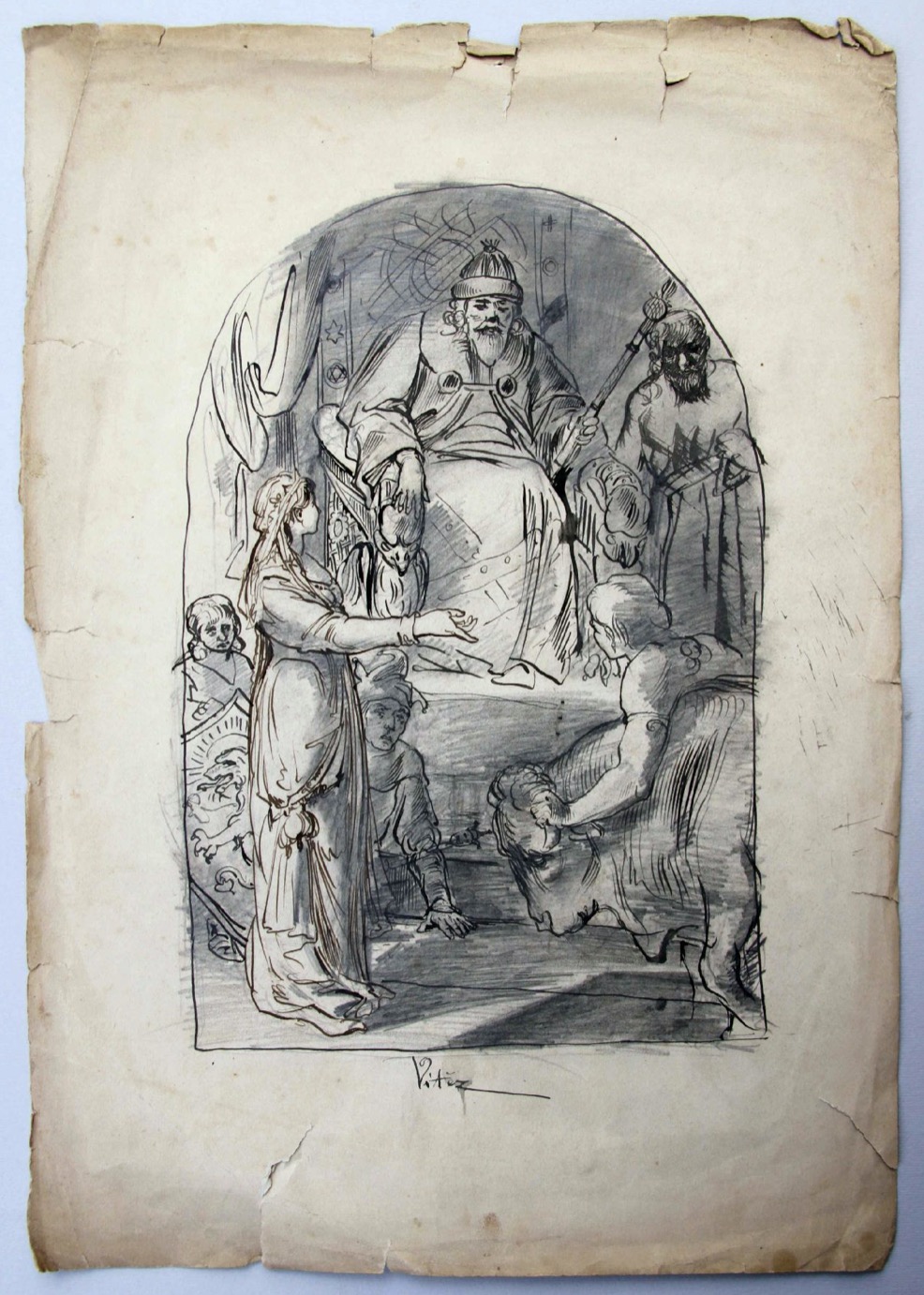This image is a detailed hand-drawn sketch on a piece of worn, yellowing parchment paper, set within an arched window. The paper appears deteriorated, with noticeable tears and dirt marks. The sketch itself, rendered entirely in black pencil, depicts a regal scene centered on an elderly king seated on a throne atop a pedestal. The king adopts a hunched posture, cloaked in a large cape and adorned with a crown, while gripping a scepter in his left hand. At his feet, there is a court jester kneeling down. To the right of the throne, an older advisor stands in a robe, positioned near a partial depiction of a bull, which a woman appears to be presenting to the king, her arms wrapped around it. To the left of the throne stands a tall woman in a long gown, extending her right arm towards the woman with the bull, as if addressing the king. Below the throne, to the bottom of the sketch, the faint cursive signature of the artist is visible.